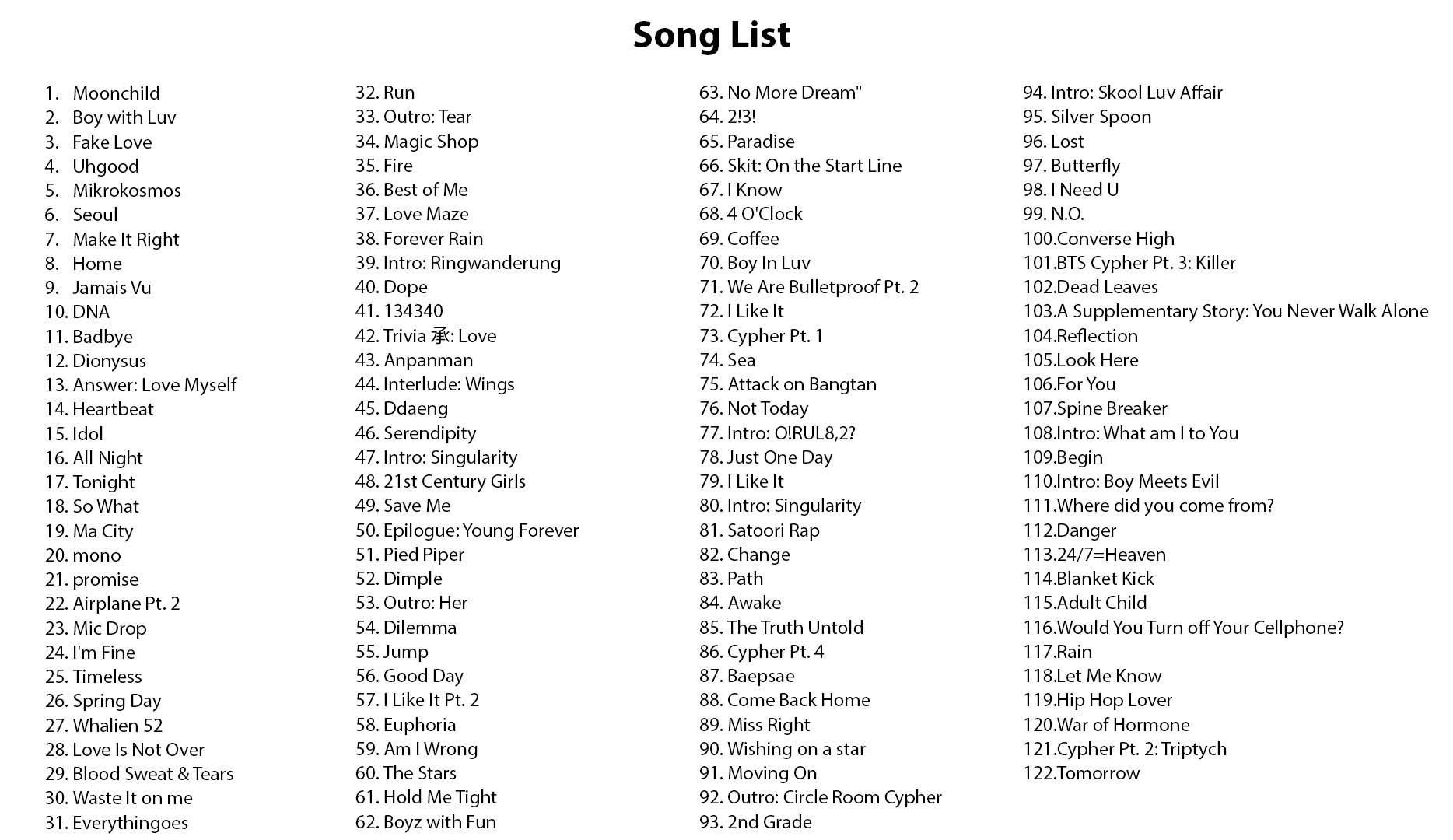This image is a screenshot of a card in landscape mode, featuring a comprehensive song list. 

In the upper left-hand corner, the title "Song List" is prominently displayed in bold letters. The card's background is a subtle off-white color, giving it a clean and classic appearance.

The list is meticulously organized into four columns, each detailing a sequential arrangement of songs by number and title:

- **First Column:** 
  - Starts with "1. Moon Child" at the top left corner.
  - Continues sequentially down to "31" at the bottom.

- **Second Column:**
  - Begins with "32. Run" at the top.
  - Extends to "62. Boys with Fun" at the bottom.

- **Third Column:**
  - Commences with "63. No More Dream".
  - Ends with "93. Second Grade".

- **Fourth Column:**
  - Opens with "94. Intro: SKOOL Luv Affair".
  - Concludes with "122. Tomorrow".

Though the list was intended to have up to 124 entries, it ultimately concludes at 122. The highlighted top 10 songs, based on preference, are:

1. Moon Child
2. Boy With Luv
3. Fake Love
4. Mikrokosmos
5. Make It Right
6. Home
7. Jamais Vu
8. DNA

This curated collection reflects the individual's preferred order of songs, despite any unfamiliarity the viewer might have with them.